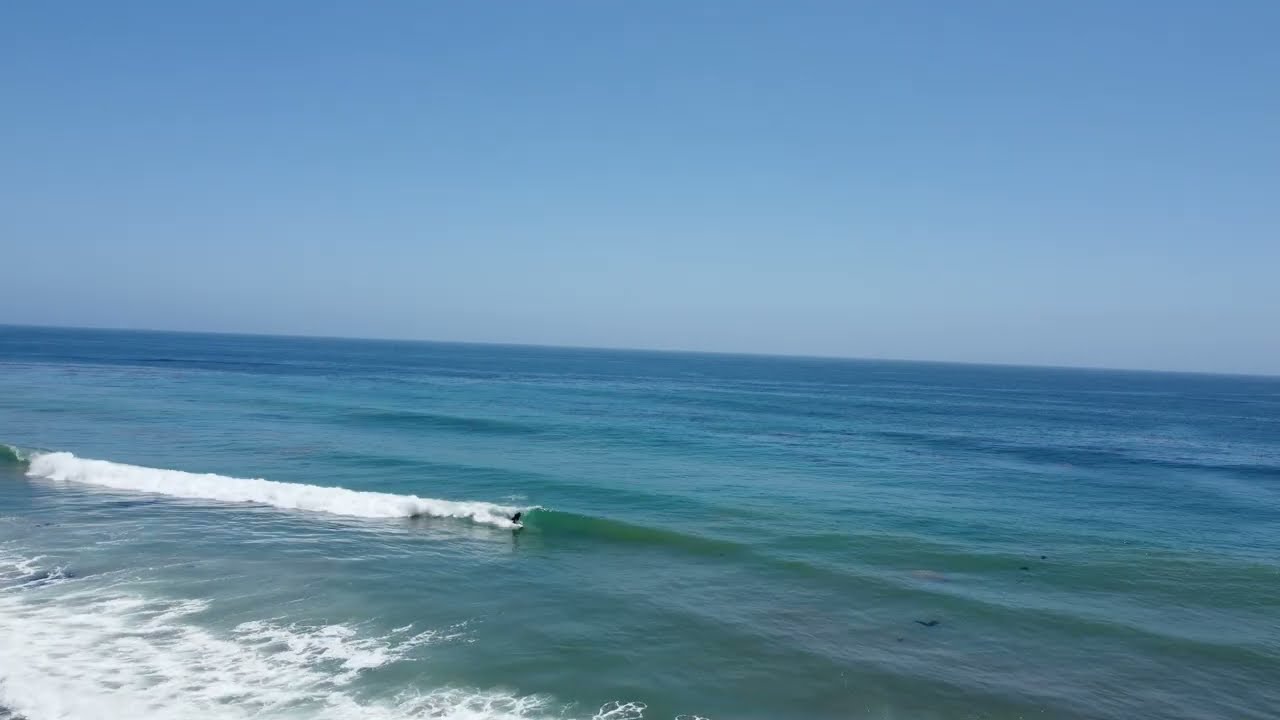A picturesque scene captured in this image shows the vast expanse of the ocean on a clear, sunny day. The top half of the photo is dominated by a flawless blue sky, devoid of clouds. Below, the bottom half displays the dynamic ocean, transitioning from a greenish hue near the shore to a deep, dark blue as it stretches to the horizon. Small to moderate waves are visible, with white foam forming on the surface where they crash. A particular focus is on a person in a black wetsuit, standing on a surfboard and riding a wave approximately 5 feet tall, situated prominently near the center of the image. Additionally, some seaweed can be seen floating on the right side of the photo, further from the surfer. The shoreline is visible with some white water marking the waves' end and a strip of sandy coast. The entire scene is slightly tilted, giving the impression it was taken at an angle.